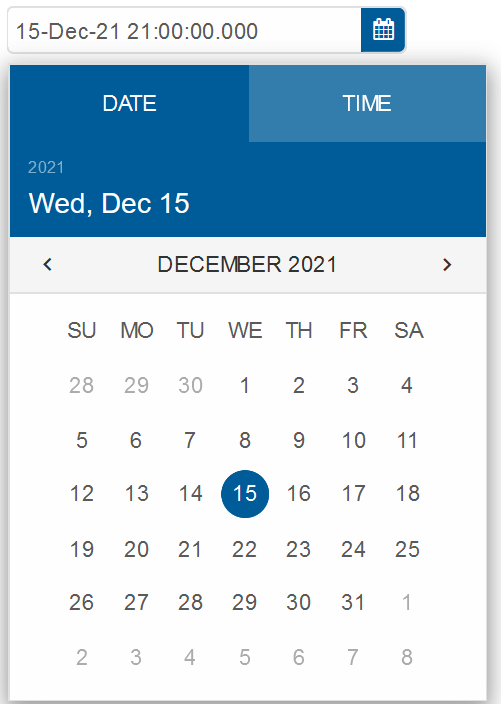A cropped screenshot of a calendar application shows various interface elements. At the top, a prominent rectangular bar spans the width of the screen. To the left of this bar is a blue icon featuring a calendar. The search bar prominently displays "15 December 21, 2100 hours.000." In the bottom left corner, a selected tab labeled "Date" is highlighted in blue, indicating it is currently active. Next to it, in a lighter blue, is a tab labeled "Time."

Just below these tabs, the year "2021" appears in small white font, with "Wednesday, December 15th" displayed in large white letters beneath it. A gray divider line separates these elements from the rest of the interface.

Centered below the divider is "December 2021" in black letters, with left and right arrows on either side to navigate through the months. Below this heading, the days and dates of the month are displayed in a grid format, with December 15th distinctly highlighted.